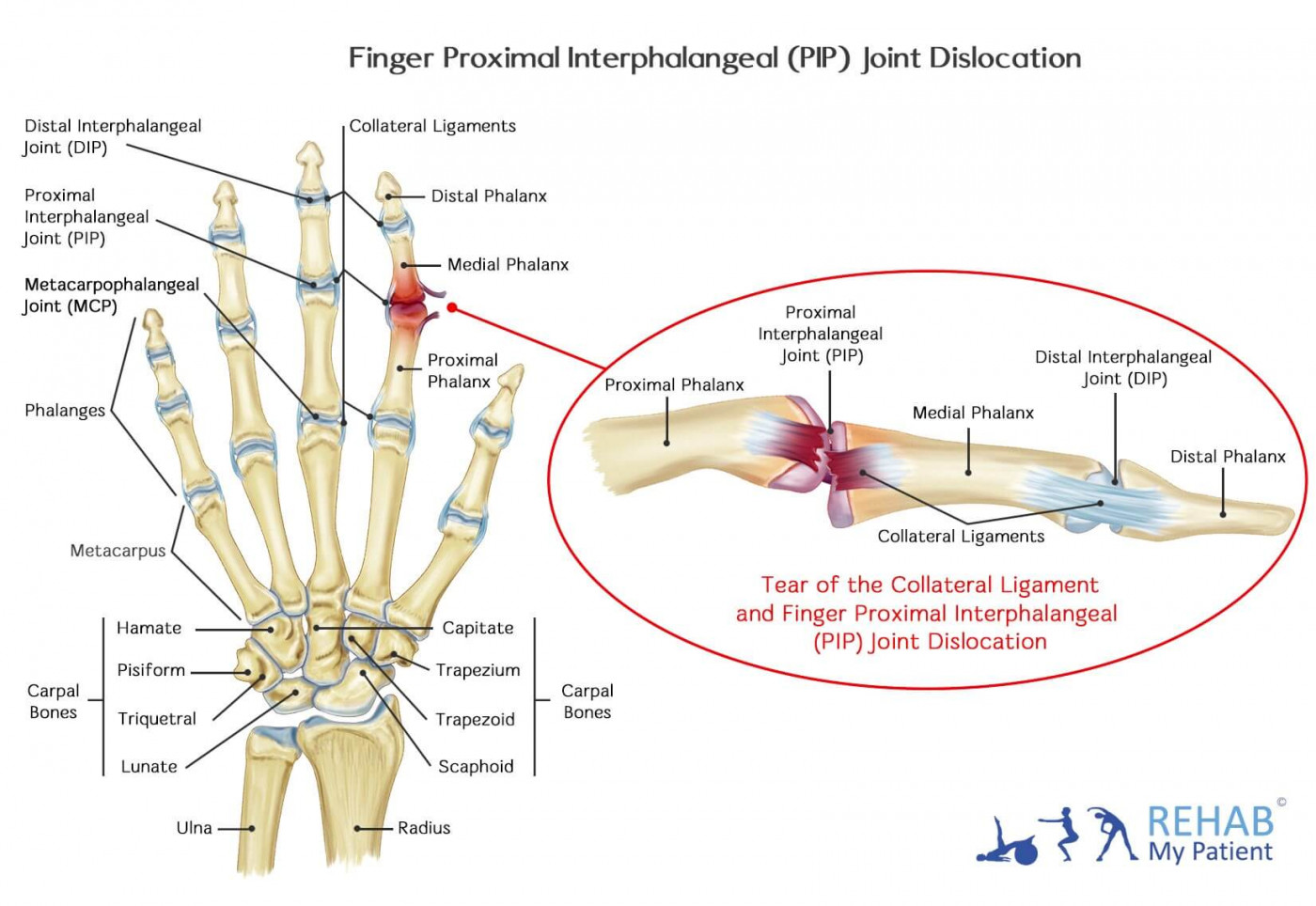**Detailed Caption:**

This diagram, reminiscent of those found in a doctor's office, is a comprehensive illustration titled "Finger Proximal Interphalangeal Joint Dislocation." In the top section, it features human stick figures demonstrating various exercises and stretches, indicating practical rehabilitation techniques. 

At the bottom left corner, the phrase "Rehab My Patient" is written in blue font. The central image displays a detailed skeleton hand, colored in shades of ivory, blue, and red. The diagram meticulously labels each part, beginning with the Distal Interphalangeal Joint, Proximal Interphalangeal Joint, Metacarpophalangeal Joints, and continuing through the Phalanges, Metacarpus, Hamate, Pisiform, Triquetrum, Lunate, Ulna, Radius, Carpal Bones, Distal Phalanx, Medial Phalanx, Proximal Phalanx, Capitate, Trapezium, Trapezoid, Scaphoid, and Carpal Bones.

Below this is another highlighted image, encircled in red, with the annotation "Tear of the Collateral Ligament and Finger Proximal Interphalangeal Joint Dislocation" in red font. This secondary diagram focuses on the Proximal Phalanx, Proximal Interphalangeal Joint, Medial Phalanx, Distal Interphalangeal Joint, and Distal Phalanx, with particular emphasis on the Collateral Ligaments depicted in ivory bone color, burgundy and pale purple muscles, and a highlighted blue muscle spot. Black lines meticulously draw attention to the specifics of each anatomical region.